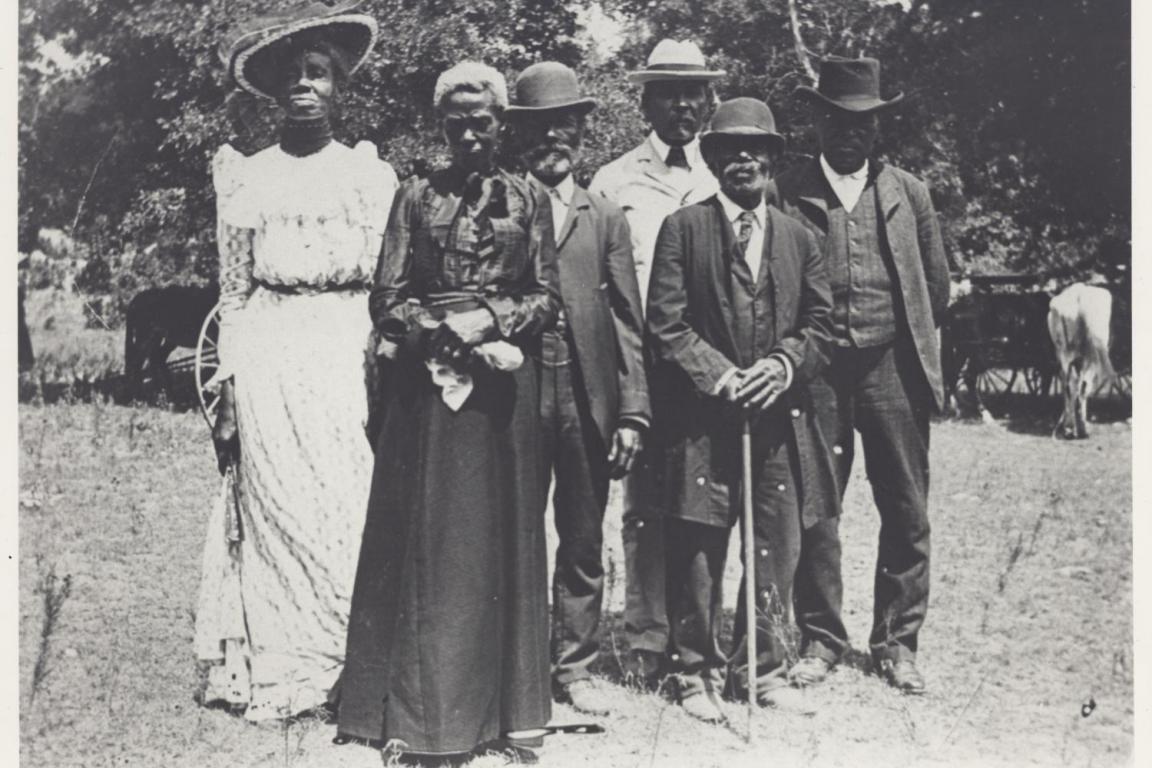This vintage black-and-white photograph captures a moment of African-American life, likely from the late 19th or early 20th century. Six individuals stand proudly in the foreground—two women and four men—dressed in their finest attire, a testament to their dignity and resilience. The men don elegant suits with long coats, ties, and a variety of hats, including top hats and bowler hats. The women wear long, beautifully crafted dresses with long sleeves; one of them sports a stylish hat. Behind them, trees frame the scene, with donkeys visible to the right and left, suggesting a rural setting. The ground they stand on is a mix of dirt and tufts of grass. This photo offers a rare and poignant glimpse into African-American wealth and fashion before the end of the Jim Crow era, celebrating a proud heritage that persisted despite the trials of the times.